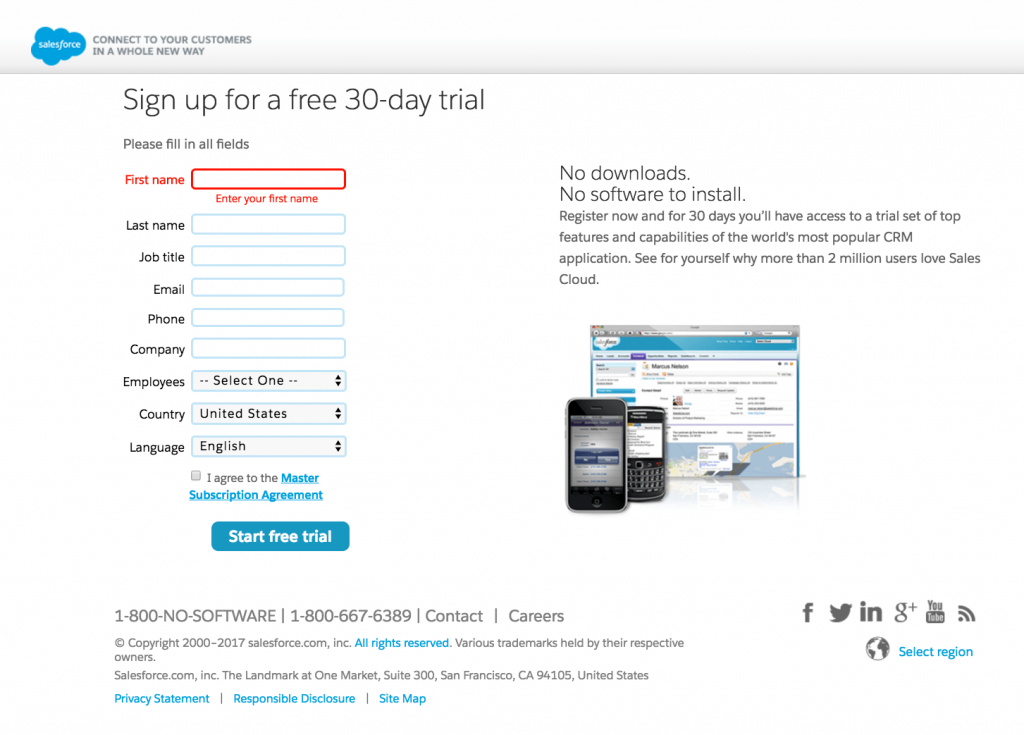Here's a detailed and polished caption:

---

Screenshot of the Salesforce Pre-Trial Sign-Up Page

In the top left-hand corner of the page, the Salesforce logo is prominently displayed, featuring white letters inside a distinct blue cloud. Accompanying the logo, a tagline reads, "Connect to your customers in a whole new way."

Centered below the tagline, a bold message encourages potential users to "Sign up for a free 30-day trial." The form below this prompt asks users to "Please fill in all fields," with the "First Name" field notably highlighted in red, indicating it is required. The form continues to list fields for "Last Name," "Job Title," "Email," "Phone," "Company," and a dropdown menu for "Employees" to select their company's size. Additional options include "Country," defaulted to the United States, and "Language," set to English.

Below these fields, there is a checkbox to agree to the Master Subscription Agreement, which must be checked to proceed. The form's footer features a prominent blue button with "Start Free Trial" inscribed in white, urging users to commence their trial.

At the bottom of the page, contact details are provided, including a contact phone number and a button for career opportunities.

---

This caption thoroughly describes the visual and functional elements of the Salesforce pre-trial sign-up page, including the layout and specific content displayed.